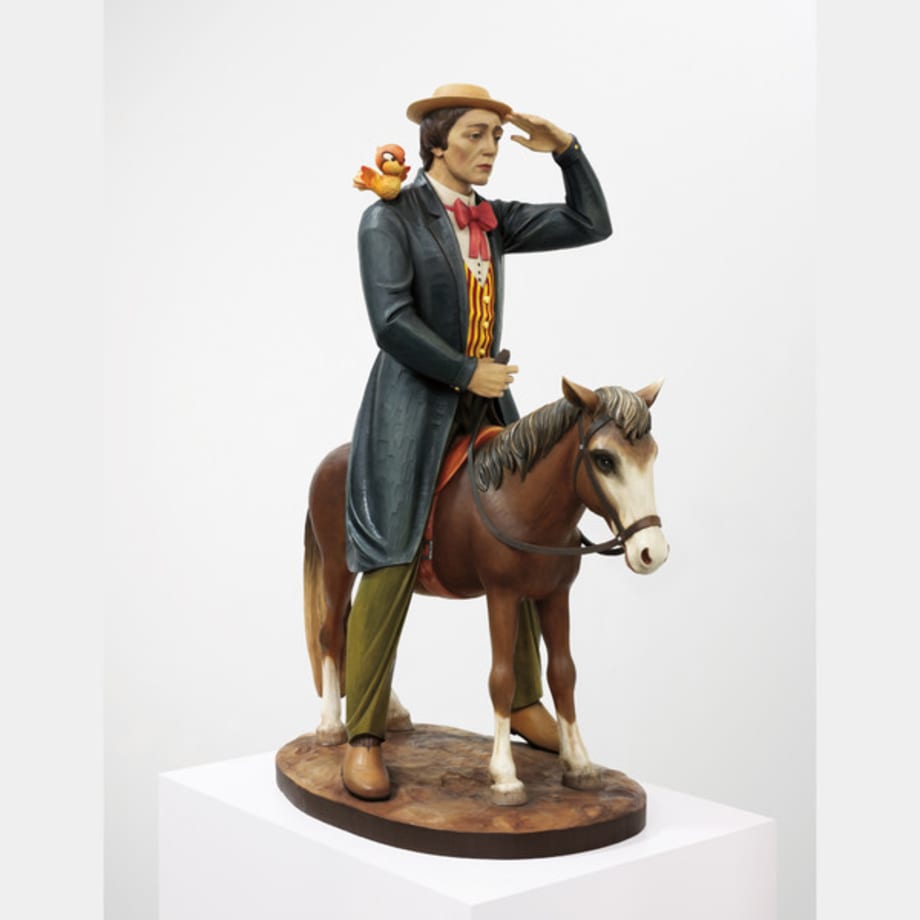The image is a vertical rectangular photograph of a sculpture by Jeff Koons portraying Buster Keaton. Buster stands astride a small brown horse with a white head, dark brown mane, and white hooves that are light brown at the very bottoms. Despite being on the horse, Buster’s feet touch the pedestal below, emphasizing the horse's miniature size. The sculpture rests on a brown base atop a white pedestal, suggesting an exhibit in a well-lit museum with white walls.

Buster is adorned in an eclectic outfit: brown shoes, green pants, a long blue jacket extending to his knees, and a white shirt coupled with a striking red bow tie. His attire includes a red and yellow striped vest and a red ribbon draped across his chest. He sports a shallow beige or straw-like hat. With a serious expression, he salutes with his right hand, while a cartoonish, orange or yellow bird perches on his left shoulder. His left hand appears to be holding the reins. The background of the image is predominantly gray, with slightly darker tones and flanked by wider white bands on either side, focusing the viewer's attention on the detailed and colorful statue.